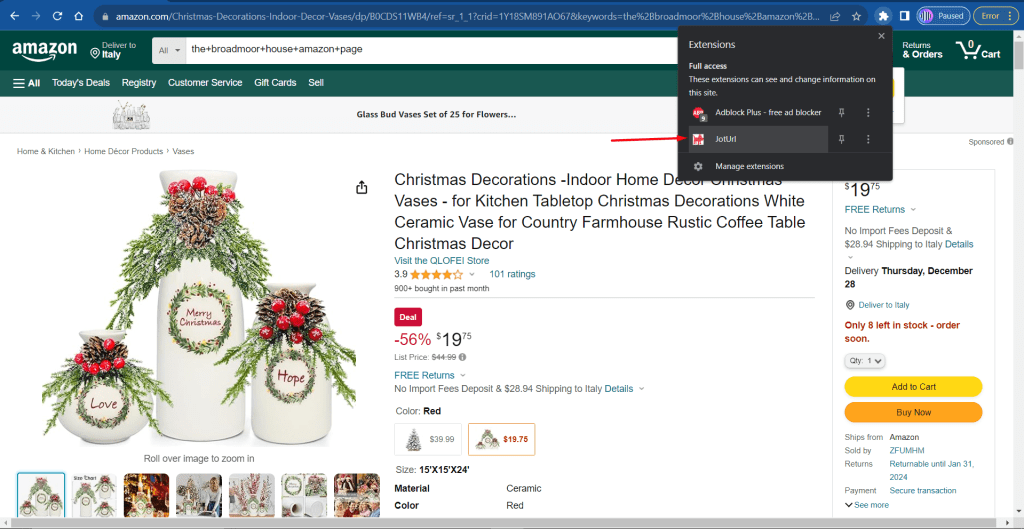This image is a detailed screenshot from an Amazon webpage taken in a web browser with a blue header at the top. In the URL bar, the address reads "amazon.com," indicating the person is browsing Christmas decorations and indoor decor specifically. To the right of the URL, a "paused" indication and an error message are visible.

The main Amazon page shows delivery options to Italy, a search bar containing the text "The Broadmoor House Amazon page," and a dropdown menu displaying browser extensions. Within this dropdown, labeled "Extensions," full access permissions for "Adblock Plus" and an unidentified extension are noted, alongside an option to "Manage Extensions."

The focal point of the Amazon page is a product listing for Christmas decorations. The image presented features ornate vases: the largest reads "Merry Christmas," while the two smaller ones are labeled "Love" and "Hope." These vases are adorned with green pine needles, tiny pine cones, and red berries. A detailed product title and a price tag of $19 are visible, alongside options to "Add to Cart" or "Buy Now."